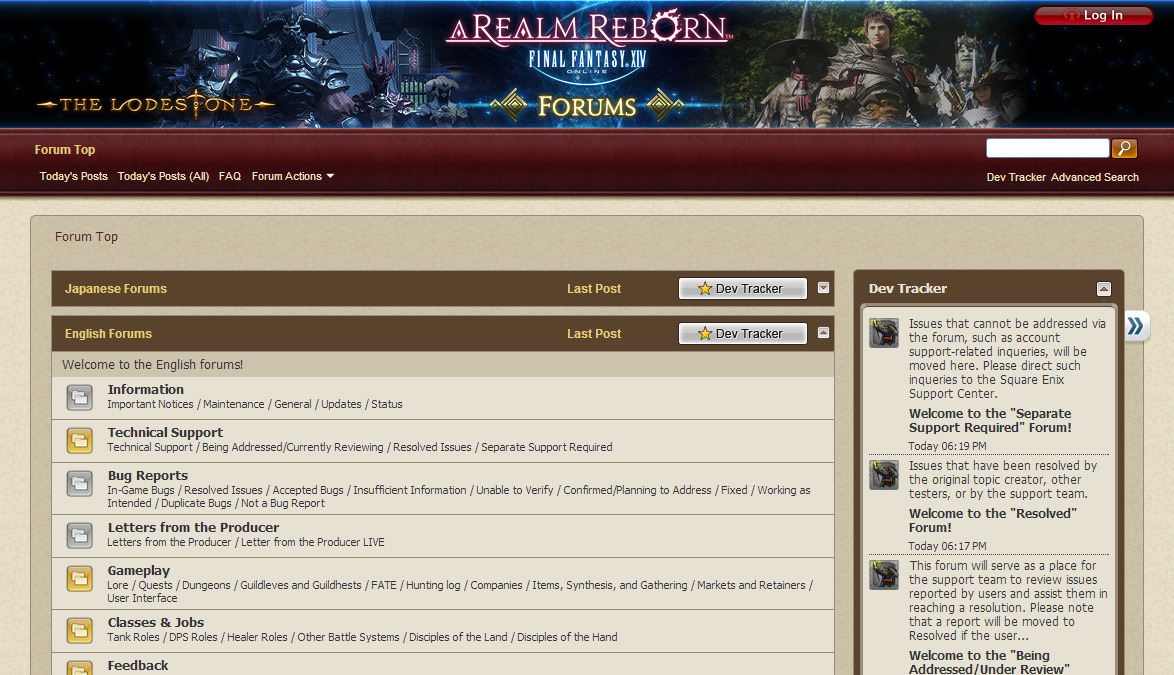A screenshot from the Final Fantasy XIV: A Realm Reborn website. At the top of the page, the title "Final Fantasy XIV: A Realm Reborn" is prominently displayed, with "Forums" written beneath it. In the top right corner, there is an option to log in. The background features a game scene with characters clad in armor wielding weapons, reminiscent of the typical dark, immersive environments found in video games.

In the forum section, "Today's Posts", "FAQ", and "Forum Actions" are listed at the top. Below that, users can choose between "Japanese Forums" and "English Forums", with a "Last Post" indicator for each section. On the right side of the page, a slender, vertical rectangle labeled "Dev Tracker" provides updates and developer posts. Meanwhile, on the left side, a welcoming message reads "Welcome to the English Forums," where users are actively typing and interacting with one another.